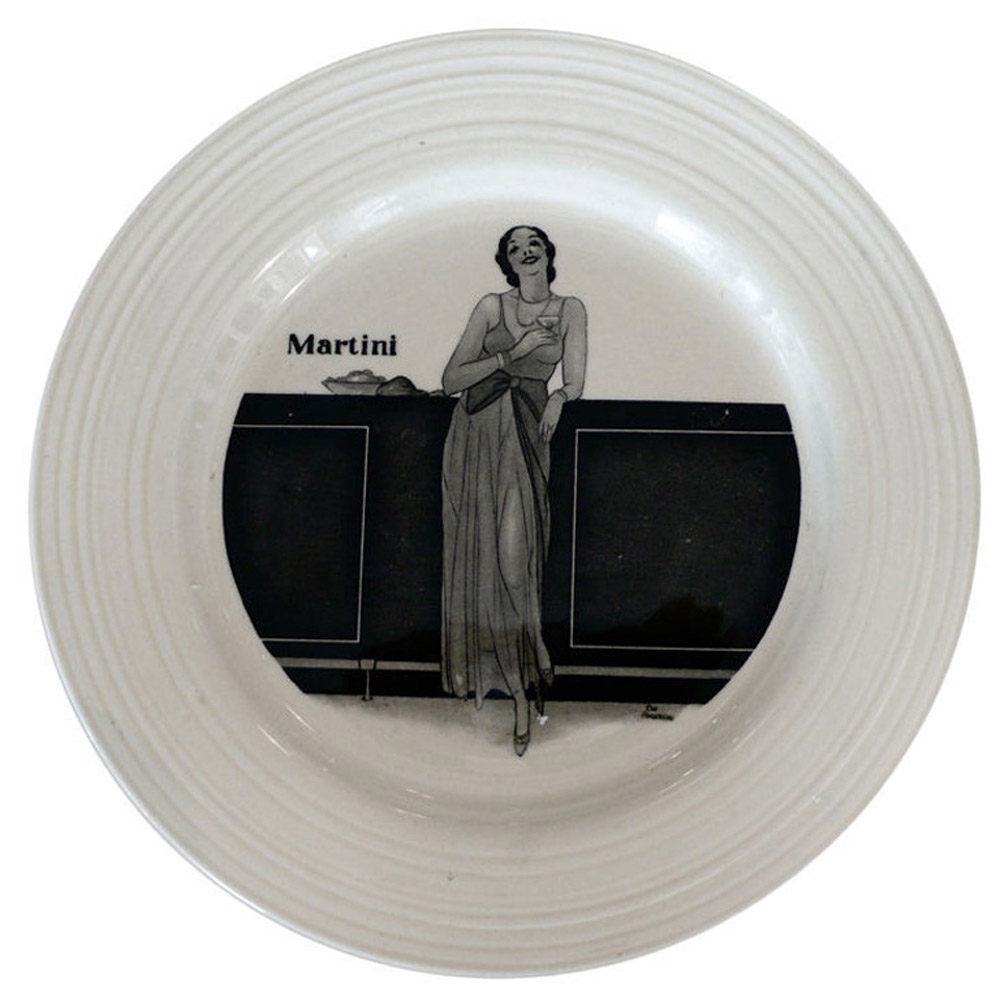This is an image of a pristine white stoneware plate with elegantly ridged edges, each ridge stretching about an inch to an inch and a half inward. Centered in the middle of the plate is a detailed black-and-white illustration of a woman exuding the style and glamour of the 1920s to 1930s. She is leaning against a dark bar, one foot on the floor and the other on a bar rail, with her elbows casually resting on the bar. The woman is flashing a charismatic smile, her hair styled in a distinctive manner appropriate to the era, flat on top and rolled on the sides, possibly set with curlers. She wears a chain necklace and a long, see-through spaghetti strap dress that flows down to her ankles, paired with high-heeled pumps. In one hand, she gracefully holds a cocktail glass, possibly a martini, affirming the word "martini" prominently written behind her on the bar. The bar also features items that appear to be food. The entire scene conveys a vintage ambiance in black and white, reflective of a bygone era of elegance and revelry.